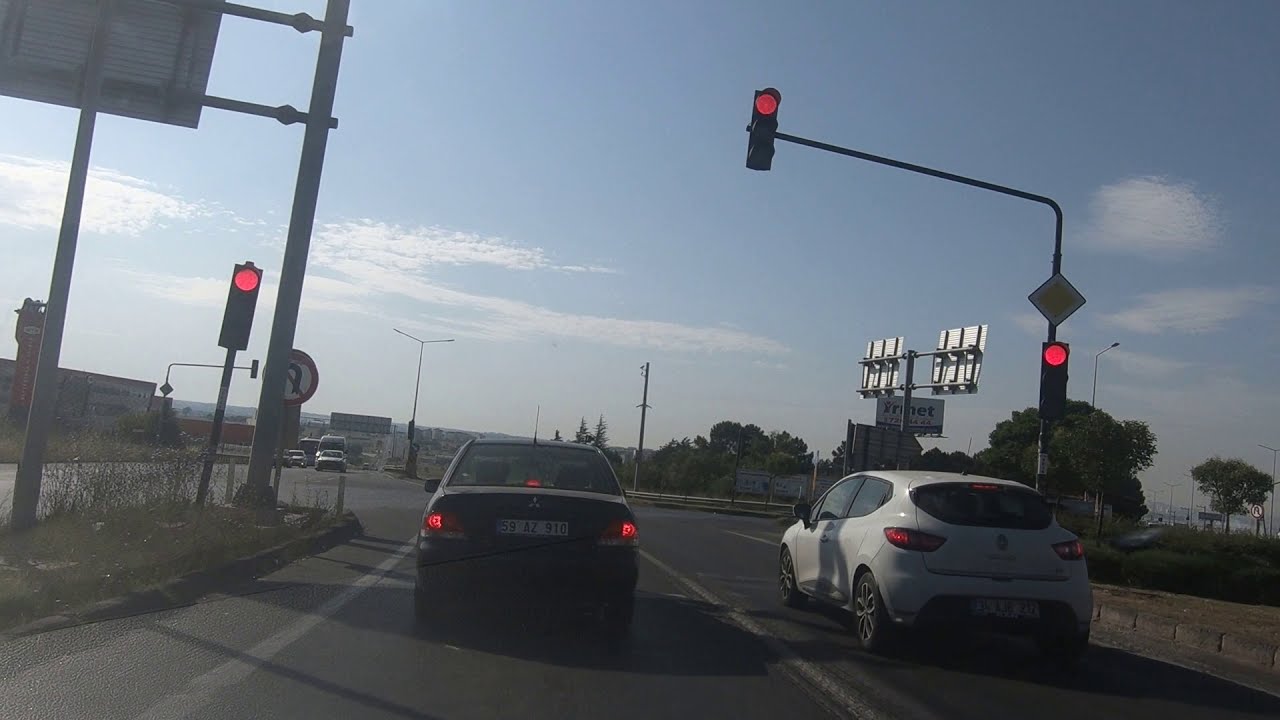The image captures a scene at an intersection where several cars are halted at a red light. Central to the photograph is a black sedan with a distinctive white and black license plate. To its right, a white car, also bearing a white and black license plate, is equally stationary. Both vehicles have their brake lights illuminated, accentuating the sense of pause and anticipation. 

The traffic is fronted by a silver pole extending over the road, supporting three red traffic lights. Additionally, there's a diamond-shaped street sign affixed to this pole. The intersection is demarcated with a prominent yellow line in the center of the black asphalt road, flanked by white lines on the road's edges. 

The sky above features a blend of light and dark blue hues interspersed with white clouds, casting a somewhat subdued light over the scene. To the left of the black sedan, another traffic light glows red, contributing to the overall halt. 

In the distant background, a few trees are visible, adding a touch of natural scenery to the urban setting. Despite the presence of white clouds, the overall lighting suggests a dimly lit environment, emphasizing the neutral and somewhat dark tone of the image.